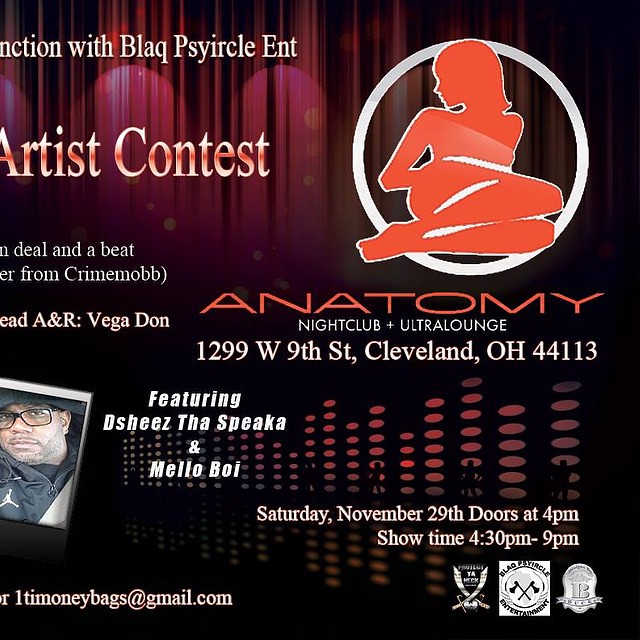The image is a square flyer advertising an event at Anatomy Nightclub Ultra Lounge, located at 1299 West 9th Street, Cleveland, Ohio, 44113, on Saturday, November 29th. The top part of the flyer features a red curtain background that transitions to black towards the bottom. The upper left corner text is partially cut off, displaying "N-C-T-I-O-N" and "black psyircle ENT," followed by "Artist Contest." The upper right corner showcases a logo in a white circle, depicting an orange silhouette of a woman sitting with her knees in front of her, looking to the side. Below the logo, bold red font spells out "Anatomy Nightclub Ultra Lounge." Prominently displayed in the bottom left corner is a photograph of a black man with black-framed glasses, alongside the names of featured artists: Dee Shees, The Speakah, and Mellow Boy. The bottom right corner states the event details: "Saturday, November 29th, doors at 4 pm, Showtime 4:30 pm to 9 pm." Additionally, there is a contact email on the bottom left: timoneybags@gmail.com, accompanied by various logos.